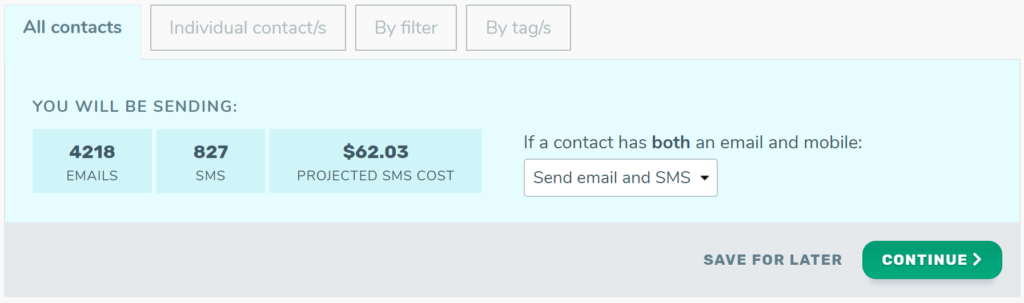This image depicts a screen from a software tool, likely an email and SMS marketing platform, displaying a detailed summary of contact management options. 

At the top of the screen, various tabs are visible, labeled: "All Contacts," "Individual Contacts," and "Contacts by Filter or Tag." The selected tab, "All Contacts," is highlighted with an aqua-colored background, indicating that the user is currently working within this section.

The primary content area summarizes the impending communication tasks. It specifies that the user plans to send communications to contacts, with the breakdown showing 4,218 emails and 827 SMS messages. Furthermore, a projected cost for sending SMS messages is provided, amounting to $62.03.

The interface also offers functionality for handling contacts with both email and mobile information, allowing the user to choose from multiple sending options via a dropdown menu.

At the bottom of the screen, a light blue bar features two action buttons: "Save for Later" and "Continue," with the "Continue" button highlighted, suggesting it's the next recommended step in the process.